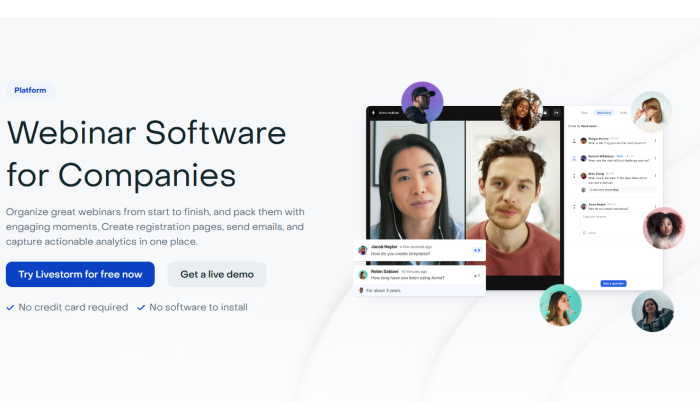This image showcases a webpage titled "Platform." On the right side, there's a screenshot resembling a Facebook or Instagram post. Depicted in the screenshot is an image featuring an Asian woman on the left and a white male on the right, surrounded by six smaller profile images encased in circles. These smaller images include one of a Black woman, one of a white woman, another Black woman, and three white women. The comment section below the screenshot is blurred and unreadable.

On the left side of the image, prominently displayed in bold text, are the words "Webinar Software for Companies." Beneath this, in smaller print, the text elaborates: "Organize great webinars from start to finish and pack them with engaging moments. Create registration pages, send emails, and capture actionable analytics in one place." Directly below this description is a blue button reading "Try Livestorm for free now." Adjacent to this button is another button labeled "Get a Live Demo." Beneath these buttons, additional text, also in smaller print, reassuringly states: "No credit card required" and "No software to install."